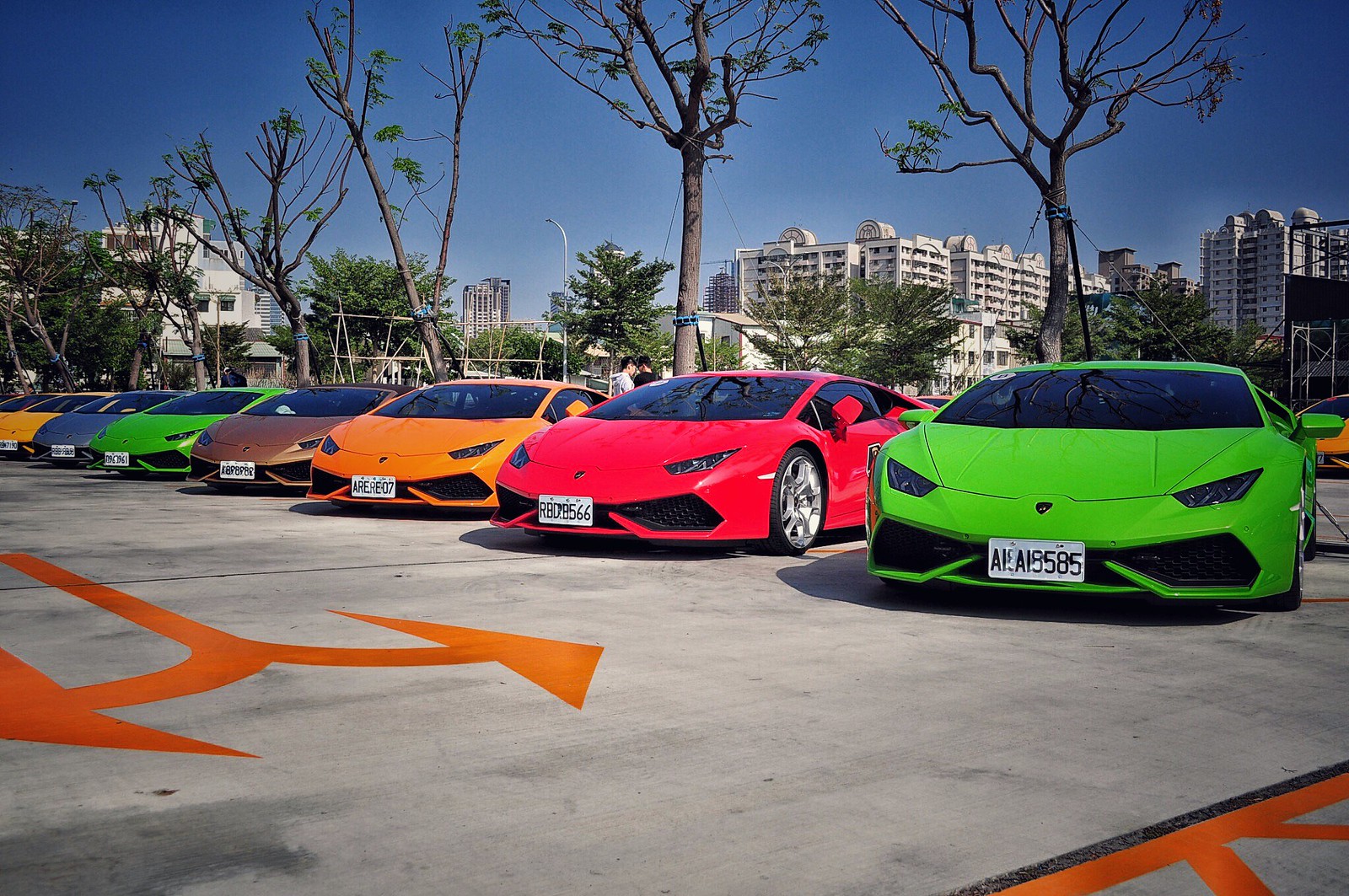In this vibrant outdoor photograph taken during the daytime, the primary focus is a row of seven high-end Lamborghinis, all parked diagonally in a concrete parking lot with bright orange directional arrows denoting the flow of traffic. The cars are uniquely colored, starting with a green Lamborghini, followed by a bright red, orange, gold, another neon green, silver, and yellow. The background features tall, white buildings resembling hotel complexes under a clear blue sky. Sparse, recently trimmed trees with minimal foliage are interspersed, adding a touch of greenery with their brown trunks and a few green leaves. A few people can be seen conversing in the background, adding a social element that suggests a gathering of car enthusiasts amidst this urban setting.